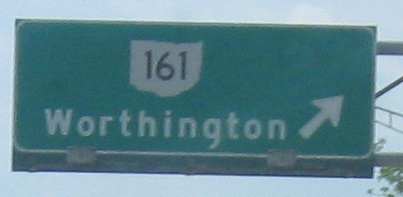This is a color photograph taken during the daytime, presumably from inside a vehicle, capturing an exit sign on the interstate. The sign is green and features the state of Ohio's outline with the numbers "161" in black inside the state shape. Below this, "Worthington" is written in white letters, accompanied by a white arrow pointing to the right. The sign is mounted on two vertical metal bars with additional cross lateral support structures. A couple of light fixtures are present below the sign, illuminating it. The sky in the background is a hazy blue with possible clouds or a dirty glass effect. The top of a tree with a few leaves is visible in the bottom right corner behind the supporting pole.